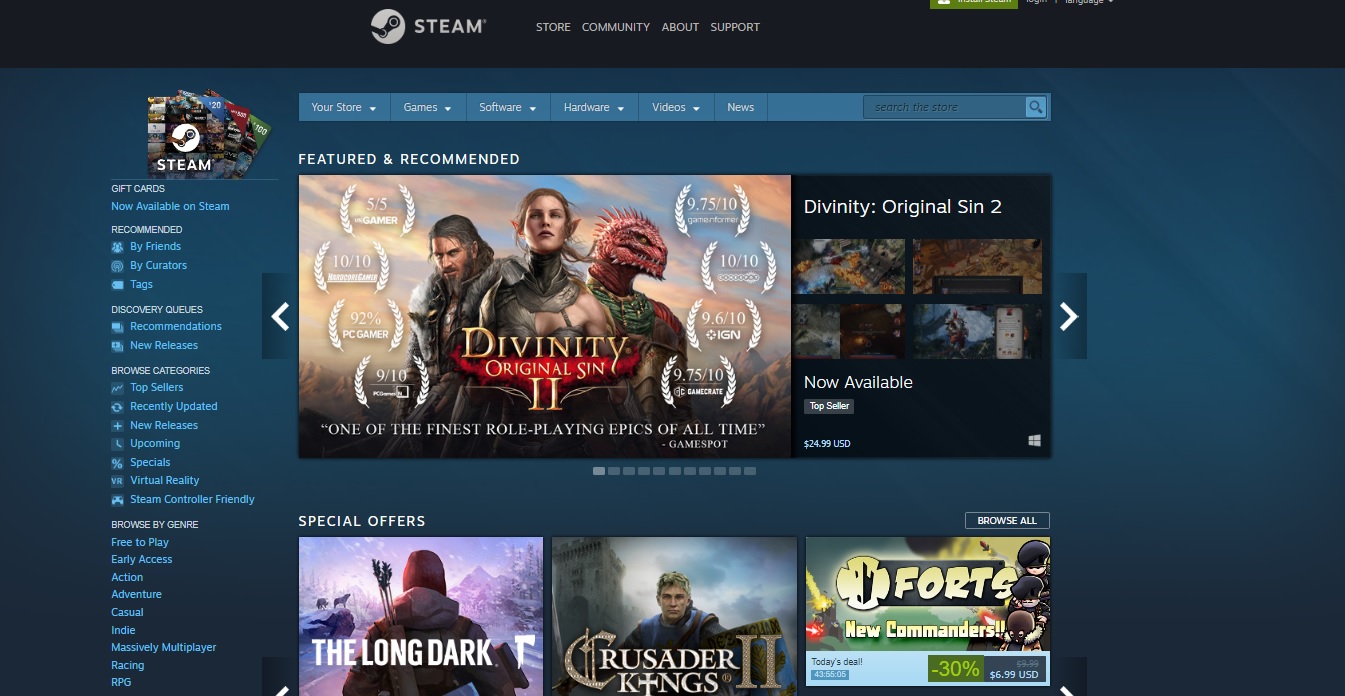This image showcases the front page of the Steam Launcher, potentially viewed through the website. Prominently featured in the upper left corner is the "Steam" name in white font, accompanied by the Steam logo—a white circular icon with a mechanical motif—positioned adjacent to the text. This logo and title sit within a dark horizontal bar, which spans the full width of the image and includes navigation tabs reading Store, Community, Above, and Support.

Below this dark bar, there is a light blue navigation menu listing categories such as Store, Games, Software, Hardware, Videos, and News. A search bar labeled "Search the Store" is also visible within this menu. 

The main content area begins with sections titled "Featured" and "Recommended." Currently highlighted in this section is the game "Divinity: Original Sin 2," prominently displayed with a collection of award symbols suggesting its high acclaim. 

Beneath this featured game, there's a section for "Special Offers," showcasing games such as "The Long Dark," "Crusader Kings," and "Forts." 

On the left side of the image, a vertical menu is discernible, though the specific contents of this menu are not detailed in this description.